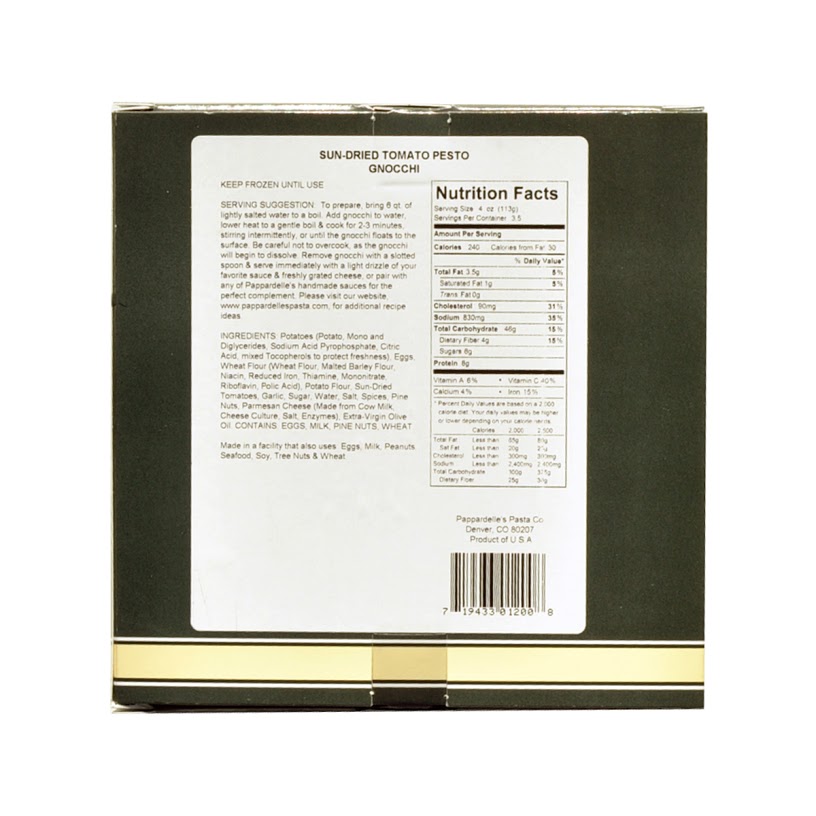The image depicts the back of a bag of "sun-dried tomato pesto gnocchi." The prominent label is white with rounded edges, and all the text on it is black. At the top, it clearly states "sun-dried tomato pesto gnocchi," followed by a note in smaller, faded letters: "Keep frozen until use." Below this, on the left, there is a serving suggestion that includes detailed cooking instructions. Adjacent to this, a rectangular box lists the nutritional facts. Further down, the label features an extensive list of ingredients and mentions that the product is "made in a facility that also uses eggs, milk, peanuts, seafood, soy, tree nuts, and wheat." Towards the bottom of the label, there's a standard barcode and additional details about the pasta company, which is named Sina Pappardelle's Pasta Company, based in Denver, Colorado, 80207, USA. The entire bag is black with a beige strip at the bottom, bordered by thin black lines, giving it a sophisticated appearance.